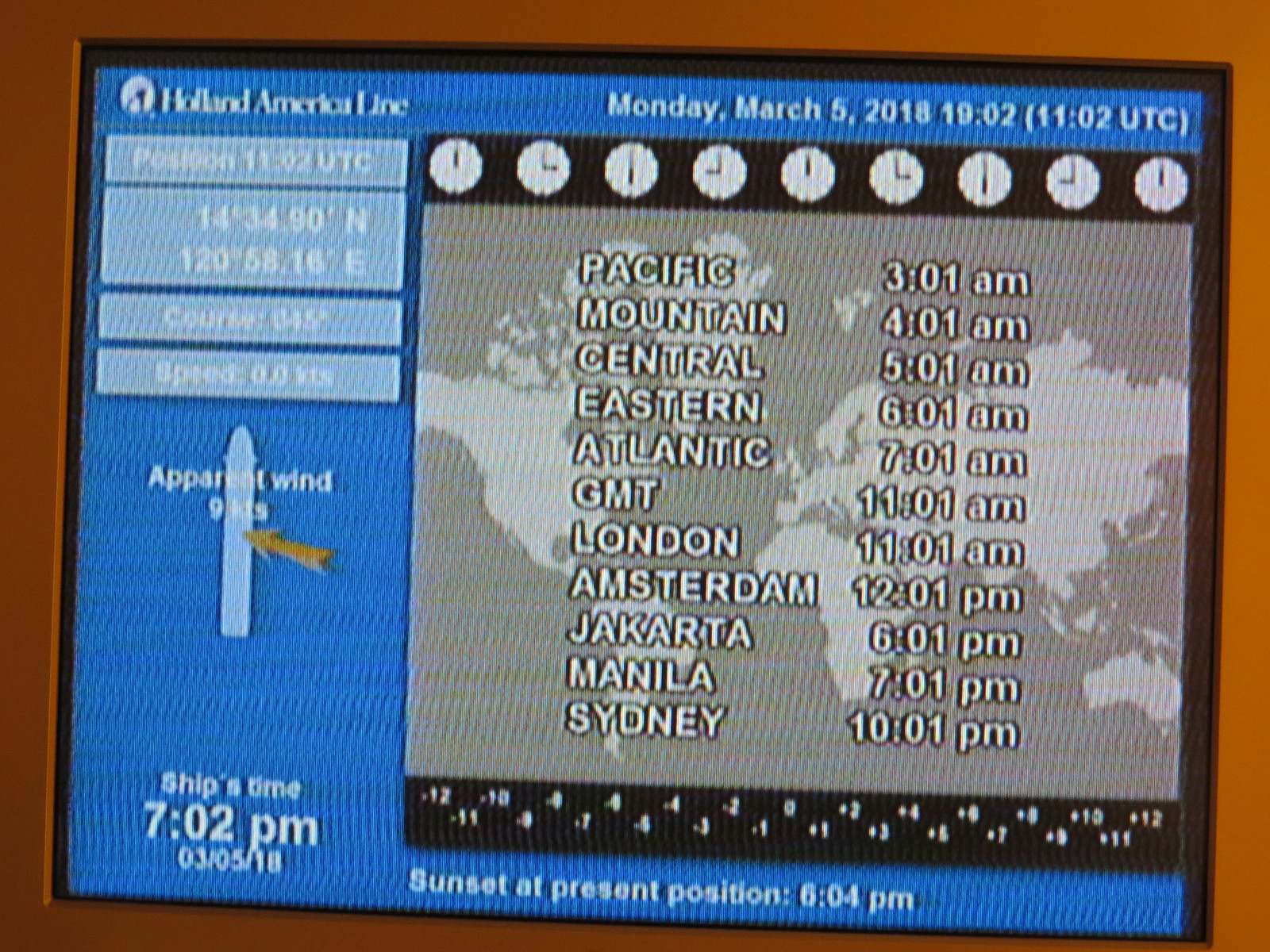The image appears to be a photograph of a digital screen displaying navigational and time-related information for the Holland America Line. The photo is somewhat unclear, as often occurs with digital images of screens, resulting in wavy distortions and pixelation. The top left corner of the screen reads "Holland America Line" and the right side shows "Monday, March 5th, 2018" with the time "1900 hours and 2 minutes," equivalent to "1100 hours and 2 minutes UTC." 

The left side of the screen includes a small blue panel with white text featuring coordinates, wind information, and speed. A silhouette of a ship is labeled "apparent wind." Below this, it notes that the ship's time is "7.02 PM," and that the sunset at the present position occurred at "6.04 PM." 

The right side of the screen is dominated by a gray and white box displaying a world map with time zones marked. Overlaid on this map are different time zones with their corresponding times: "Pacific 3.01 AM, Mountain 4.01 AM, Central 5.01 AM," etc., alongside other listed time zones like "Eastern, Atlantic, GMT, London, Amsterdam, Jakarta, Manila, Sydney." At the top of this section, there are crude clock faces indicating current times in these zones. The screen itself is framed with brown borders, adding to the sense of an on-board navigational interface.